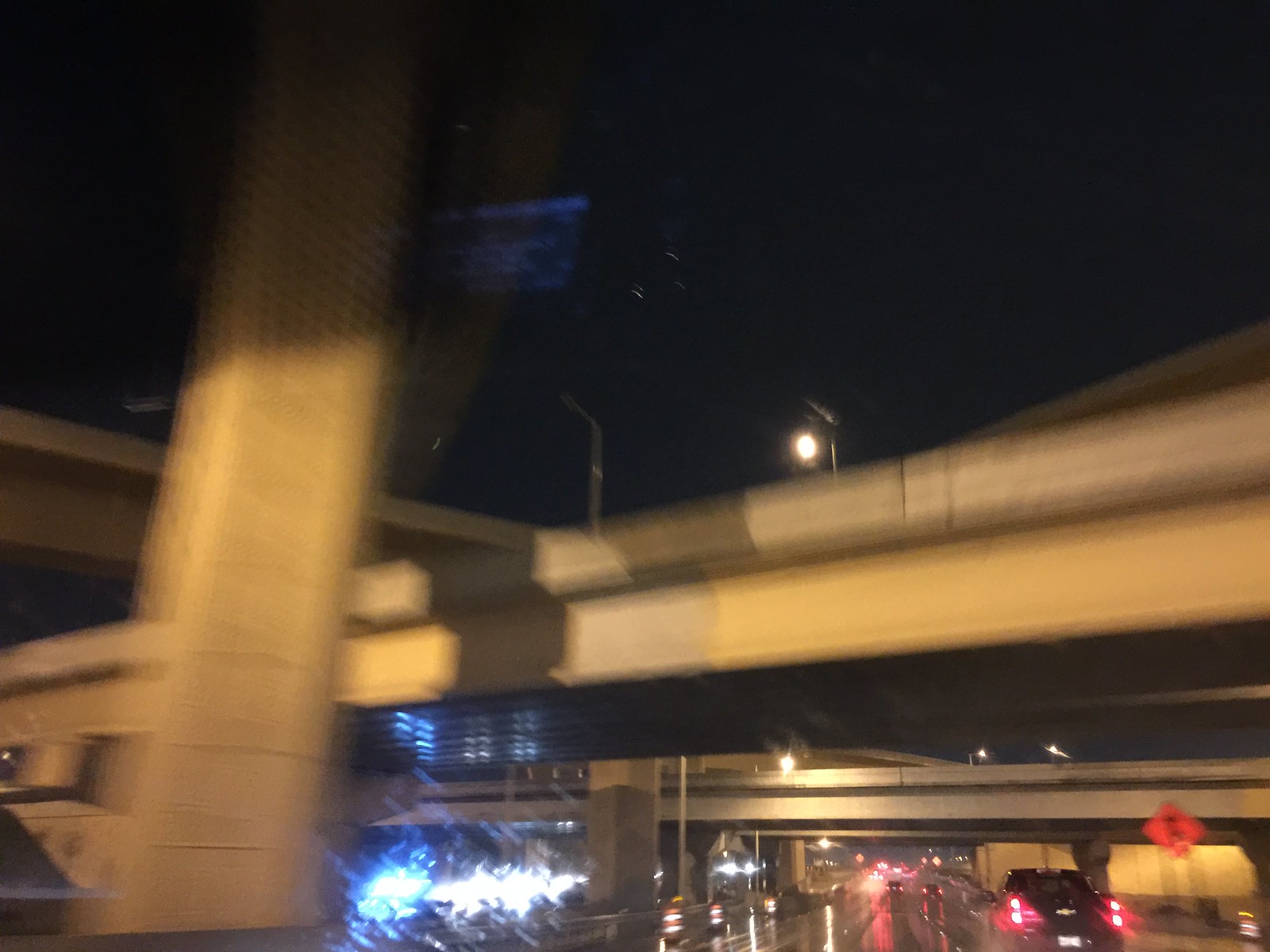Photograph Description: 

This night-time photograph, wider than it is tall, captures the view from inside a car stuck in traffic. The exact moment is after a recent rainfall, evidenced by the glistening, slightly wet road surface. Dominating the scene are the intricate concrete overpasses, illuminated by the blur of red taillights from the cars ahead. A substantial overpass stretches horizontally from left to right, complemented by additional overpasses layered in the background. On the left side, a vertical concrete pylon rises from the bottom to the top of the image. The blurry lights from potential storefronts on the left, emitting white and blue hues, add to the urban ambiance. Further, a tall structure, possibly a building or a parking garage, looms in the background, partially obscured by the overpasses. The scene encapsulates the essence of a rainy night in the city, complete with reflective surfaces and the static congestion of traffic.